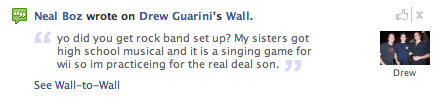The screenshot depicts a social media post. On the left side, Neil Bose wrote on Drew Guarini's wall, asking, "Yo, did you get a rock band set up? My sister's got High School Musical and it’s a singing game for Wii, so I'm practicing for the real deal, son." Below this text, there's an option labeled "See wall to wall.” The background is white. On the right side of the post, there is a slightly blurry picture of three men standing and posing together. Below this photo is the caption, "Drew." Above the picture are like and X symbols.